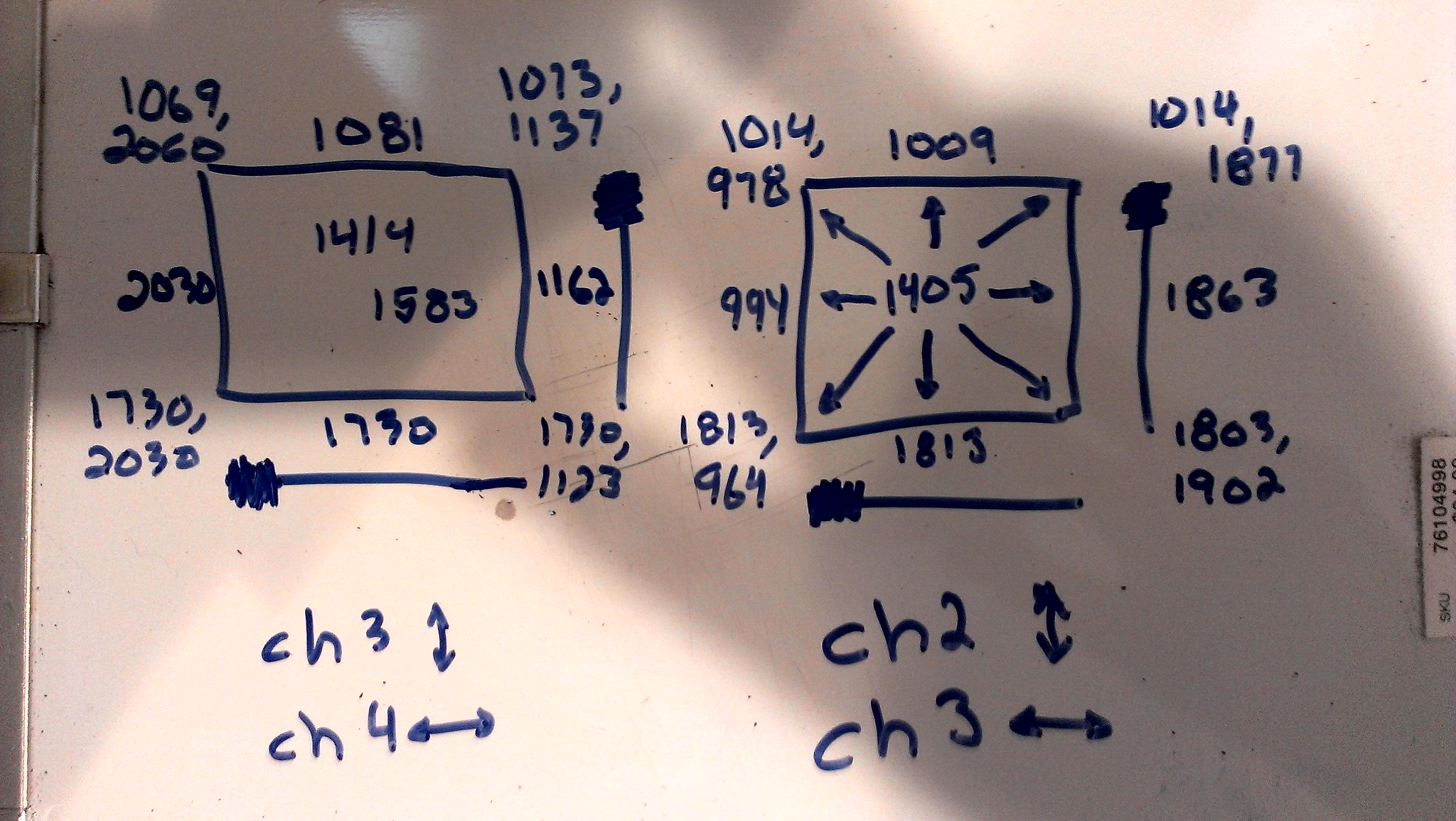In this image, a piece of light orchid-colored paper with black print is prominently featured, secured on the side by a small silver clip. Situated at the very far right-hand corner of the paper is a small white tag adorned with a series of black numbers. 

The paper itself is divided into two distinct squares. Within the first square, the numbers 1414 and 1583 are displayed prominently, while above this box, the numbers 1069, 2060, 1081, 1073, and 1137 are listed. On the right side of this square, the numbers 1162, 1730, and 1123 are written, and at the bottom, the number 1730 appears once more. To the left, the numbers 2030, 1730, and again 2030 can be seen, accompanied by a dark spot intersected by a straight line.

The second square includes the number 1405 and is marked by arrows pointing in multiple directions. At the bottom of this square, the annotations "CH3" with arrows pointing up and down, and "CH4" with arrows pointing left and right, are visible. Below this square, on the right side, the letters "CH2" are accompanied by arrows pointing up and down, and "CH3" with arrows pointing left and right.